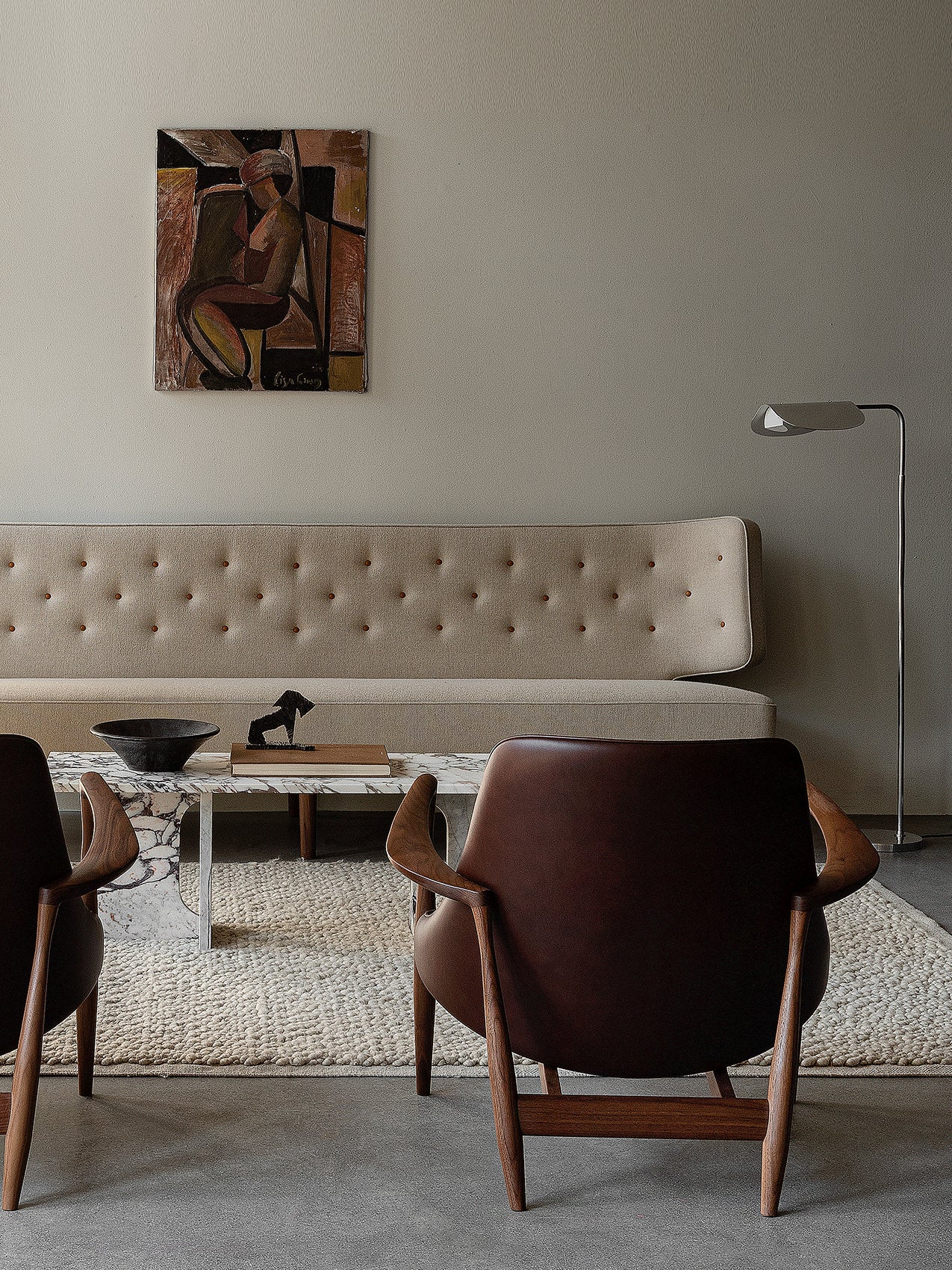The image depicts a simple, clean room with modern decor. The focal point is a long beige couch with clean lines, positioned against a white or off-white wall. Above the couch, a modern painting in brown and black hues, with a cubist influence, adds an artistic touch. Beneath the couch is a fluffy white or beige rug, adding a cozy element to the space. Centralized in the room is a black and white coffee table with a marble-like design. On the table, there is a brown book, a small statue of a dog, and a black bowl. In the foreground, the backs of two brown leather chairs with a brown frame are visible, the one on the right side fully seen, while only part of the one on the left is visible. A lamp is positioned on the side of the room, providing additional light. The wall in the background also displays subtle slate gray shades, enhancing the modern and minimalist aesthetic of the space.